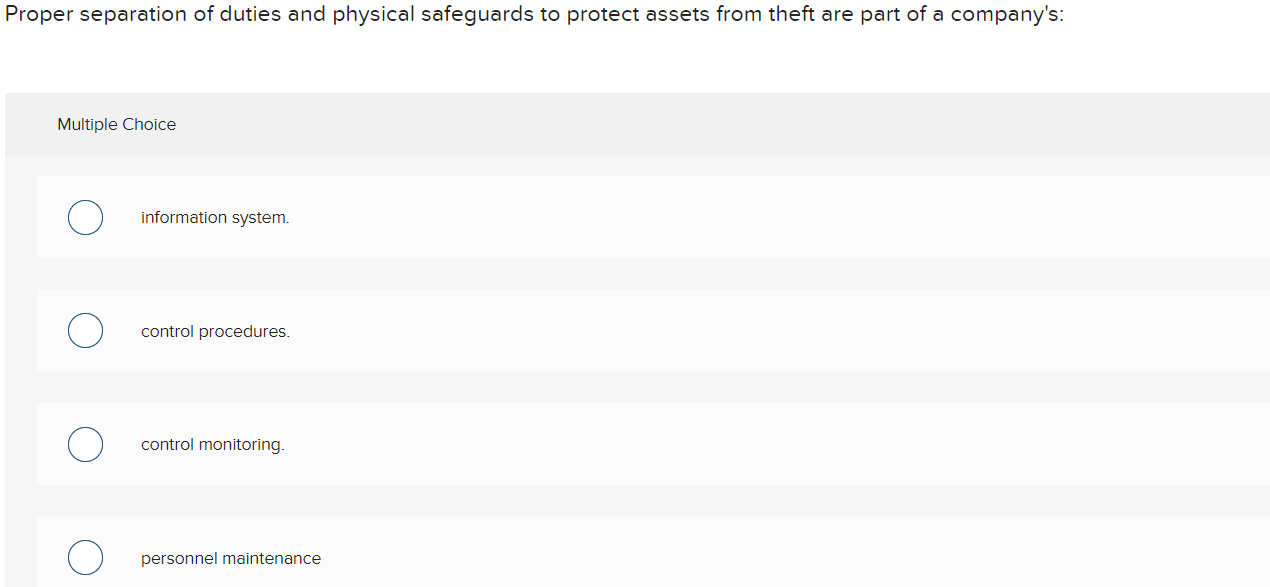This rectangular image, featuring a gray background, appears to be a screenshot or photograph of a test question, likely from an exam or study material. At the top of the image, the test question reads: "Proper separation of duties and physical safeguards to protect assets from theft are part of a company's." Below this question, there are four unmarked circles indicating multiple-choice answer options. 

The first answer option, highlighted with a light gray background, is labeled "information system." Following this, the second unmarked circle is accompanied by the text "control procedures." The third unmarked circle has the label "control monitoring," and the fourth and final unmarked circle is paired with the text "personnel maintenance."

Aside from the text and the four unmarked circles, there are no additional elements or graphics on the page. The image is distinctly wider than it is tall, emphasizing its rectangular shape.